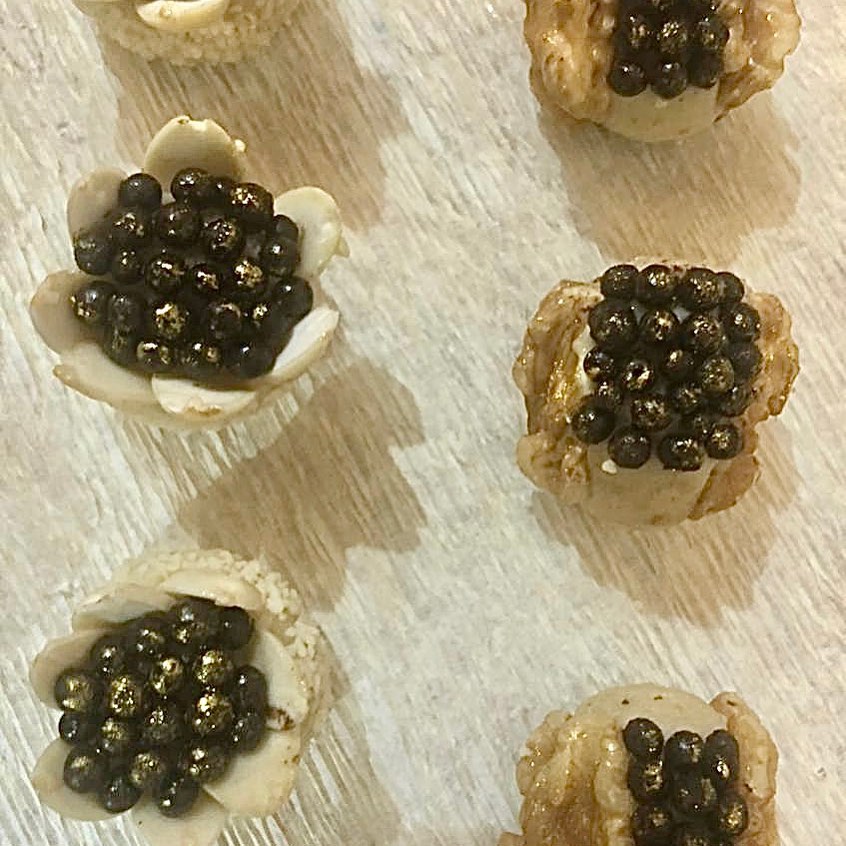This photo captures a close-up view of an artistic arrangement that blends culinary and decorative elements, arranged on an off-white surface. The image showcases six objects, though some are partially cut off from view, with three fully visible and two more partially on the right side. Each object appears to be composed of multiple small, black spheres, possibly resembling caviar or tapioca pearls, with a dusting of gold flakes. These spheres are centrally placed either atop a flower-like base or embedded within a rock-like structure. Two of the items on the left have a petal-like base, reminiscent of a flower, with the black spheres nestled in the center, giving them an ornate, decorative appeal. The other objects on the right, while lacking petals, feature the same black, gold-dusted spheres, set against a solid, golden-brown base with slightly scalloped edges, bearing a resemblance to mineral formations. The distinct textures and colors create a visually striking composition that blurs the line between edible delicacy and art piece.